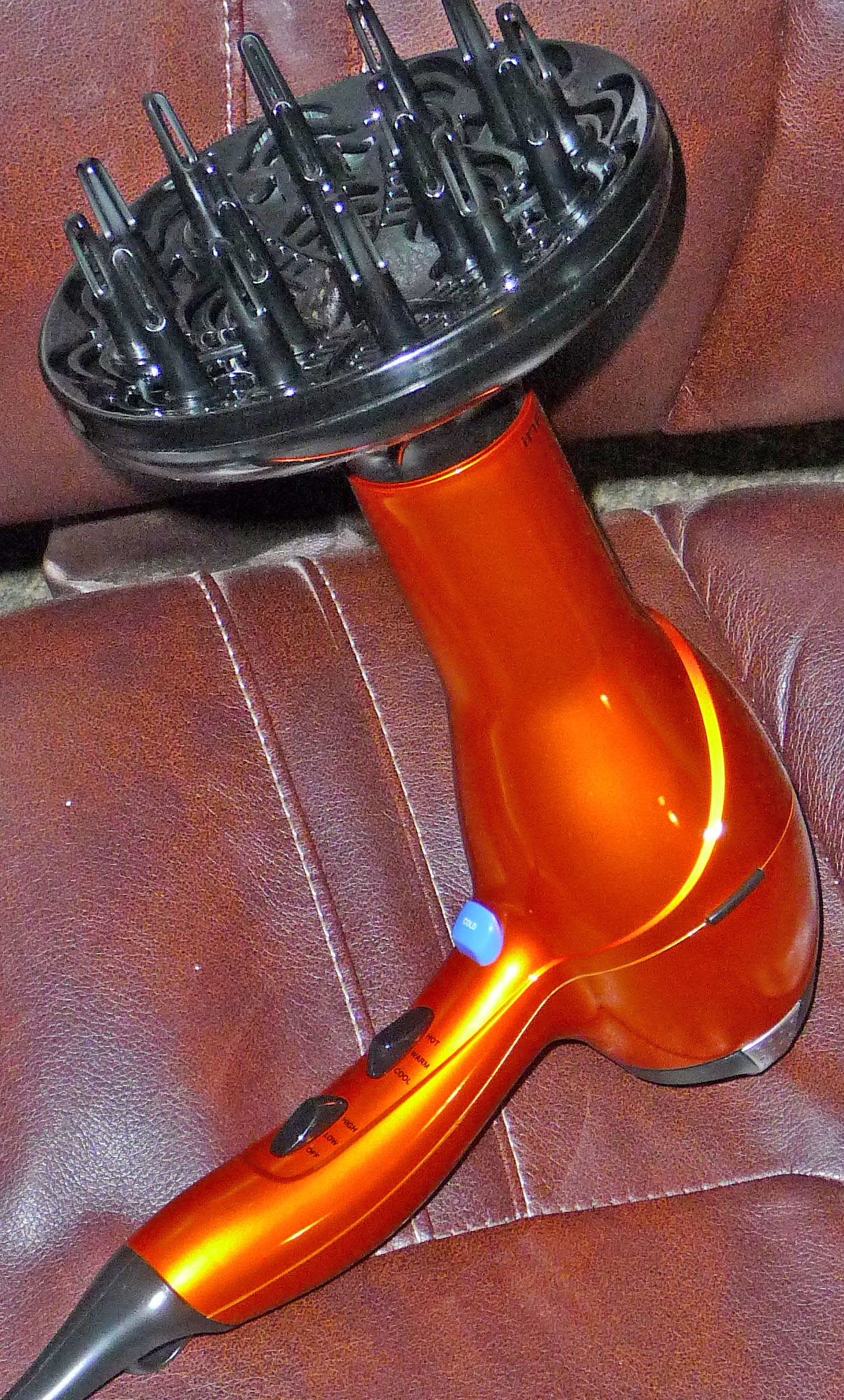The image depicts a detailed and vibrant hairdryer resting on a piece of dark, brownish-red leather furniture, possibly a sofa. The hairdryer is predominantly a hot, shiny orange color with a coppery-orange handle, body, and barrel. Around the body and extending down the handle, a yellow highlight accentuates the design. The handle features three controls: two black rocker-style switches with three positions and a blue button near the base with white lettering. The base of the handle where the cord connects is black.

The hairdryer is fitted with a black, circular diffuser attachment at the end of the barrel. This dish-shaped diffuser has many openings and sports concentric rings of small, black pillars or fingers extending from its surface, likely designed for styling hair. The hairdryer lies with the barrel pointing up at an 11 o'clock angle, showcasing both its utility and aesthetic appeal on the reddish-brown leather seat, with a visible separation between the top and bottom cushions of the furniture.